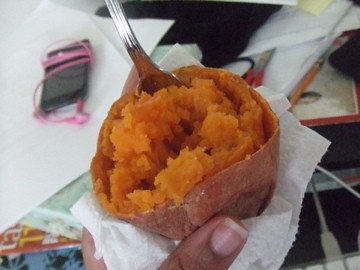This detailed photograph captures a cluttered tabletop scene featuring a mixed-up, half-cut sweet potato held in a white napkin or paper towel, with a metal spoon sticking out of its fluffy orange interior. A person's thumb, slightly elongated, is visible near the bottom of the image, holding the napkin. The bottom right corner shows the edge of a computer keyboard with white keys and a gray cable. Accompanying the keyboard is another white cable leading beneath the napkin. In the background, we see a variety of items: a red piece of paper with a yellow pencil on top, mailing envelopes, and additional papers. To the left of the napkin, a smartphone with a pink earbud cable wrapped around it lies atop the papers. Partially visible at the top left, there is also a pair of scissors with red handles. The entire scene conveys a mix of work and snack break chaos, with the sweet potato being the central focus amidst everyday clutter.